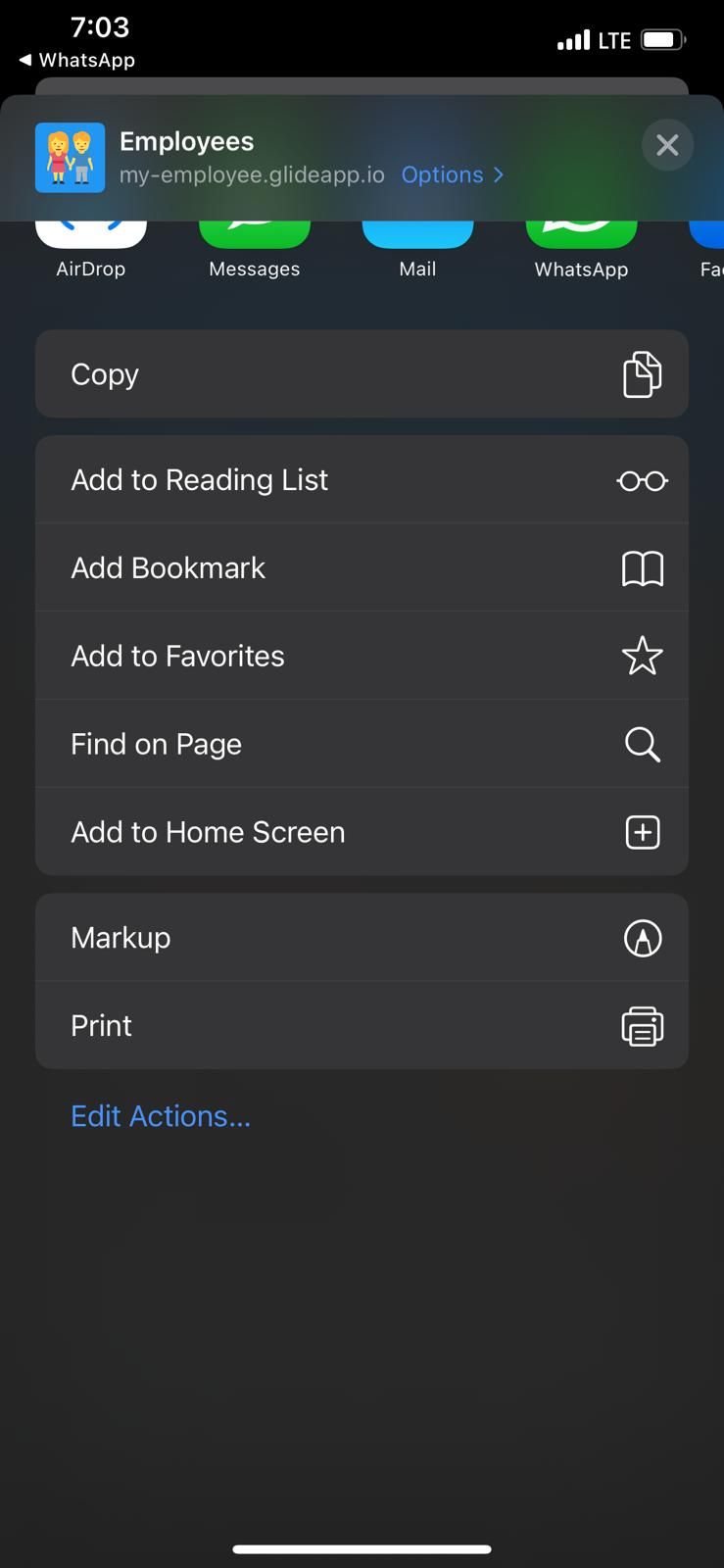The image captures a smartphone screen with a dark interface overlay at the top. In the dark status bar, the time "7:03" is displayed on the left, alongside a notification that says "WhatsApp." On the right side of the status bar, there are four signal bars labeled "LTE," and a battery icon that is nearly full.

In the background, several app icons can be partially seen: a white icon labeled "AirDrop," a green icon labeled "Messages," a light blue icon labeled "Mail," another green icon labeled "WhatsApp," and an additional blue icon whose label is obscured. 

A mostly opaque dark gray pop-up box covers part of the screen. On the left side of this box, there is a blue square containing a cartoon image of two people with the label "Employees." Below this, it says "My-Employee.glideapp.io" in small print, followed by a blue hyperlink labeled "Options." In the upper right corner of the box, there is a circle with an "X" in it, indicating a close button.

The pop-up includes several options: a box that says "Copy" with a clipboard icon to its right, another box below it labeled "Add to Reading List" featuring a glasses icon on the right, and a third option at the bottom left that says "Add Bookmark."